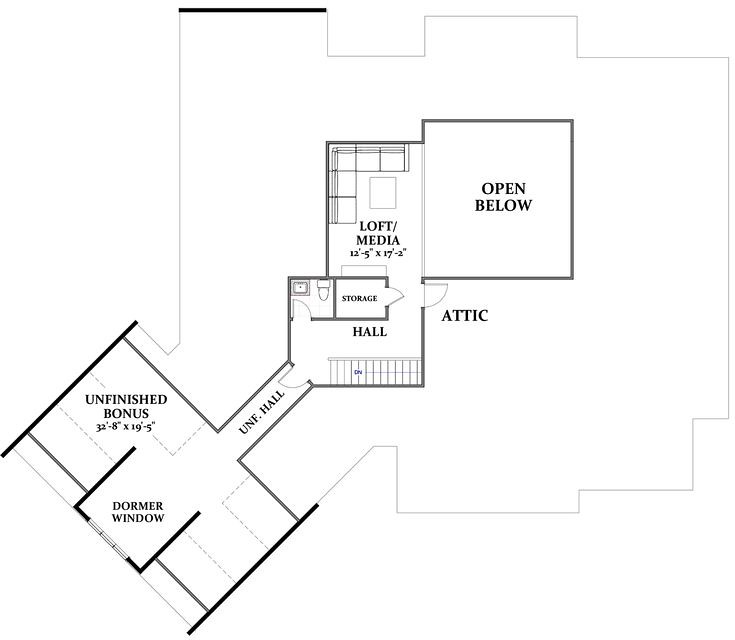This illustration appears to be a floor plan with detailed annotations. In the lower left corner, there is an area marked as "unfinished bonus," followed by dimensions "32-8 by 19-5." To the right of this, bold black text labels a "dormer window." Moving upwards, a long rectangle labeled "UNF.HALL" leads into a square area marked "hall." Directly above this hall is a box indicating "storage," adjacent to drawings resembling a toilet and sink, suggesting a bathroom area. Above the storage section, the text "loft/media, 12-5 by 17-2" is noted, with some 3D squares appearing in the upper left corner of this space. To the right, a larger square is labeled "open below" in bold text, with "attic" written beneath it without any bounding square. Encasing the entire layout is a large square outline that dips down and rises up, encompassing the other elements in the floor plan.